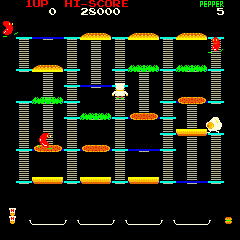This image is a screenshot from an 8-bit video game, reminiscent of the classic arcade style typified by Donkey Kong, though it is a different game. The structure of the game screen is a square tower-like construct with ladders placed at various points, connecting different levels of the tower. 

In the center of the image, a character is seen climbing up a ladder. There are various elements scattered throughout, including a snake and a cloud-like object. The game features food items as obstacles or targets: the top level holds burger buns, the middle section includes layers of lettuce and meat patties, and the bottom level has another set of burger buns. These layers are connected by ladders on which the player can move.

In three of the four corners of the screen, there are different figures, possibly enemies or other characters. The top portion of the screen displays game information including a "1 UP," a "High Score" label, "Pepper" with the number five next to it, and a current score of 8,000 points.

This game has strong associations with 1980s Nintendo titles, though the exact name escapes immediate recollection. The combination of climbing ladders, avoiding enemies, and interacting with food items provides a nostalgic glimpse into the vintage 8-bit gaming era.